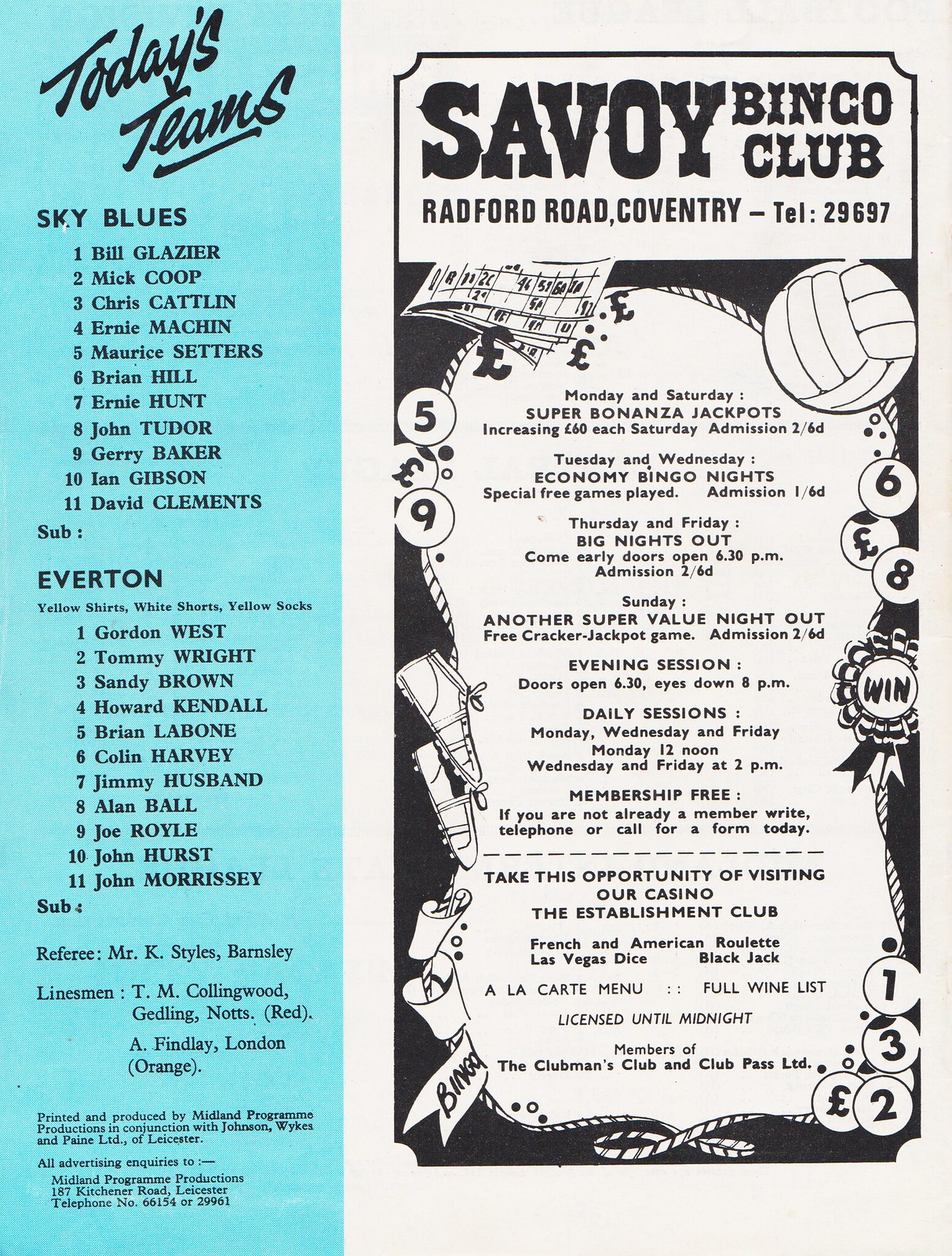The image is a piece of paper divided into two sections. On the left, printed on a light blue background, is a soccer program listing the teams and players for an English soccer game between Coventry, referred to as the Sky Blues, and Everton. Each team's players are numbered 1-11 in black text. Below the team rosters, the names of the referee and linesmen officiating the game are listed. On the right side, against a white background, there is an advertisement for the Savoy Bingo Club located at Radford Road, Coventry. The advertisement features black text and showcases bingo balls and game-related icons. It provides details about various bingo sessions: Super Bonanza Jackpots on Monday and Saturday, Economy Bingo Nights on Tuesday and Wednesday, Big Nights Out on Thursday and Friday, and a Super Value Night on Sunday. It also includes information about admission fees, membership details, and encourages visiting their casino, The Establishment Club, offering contact methods for more information.